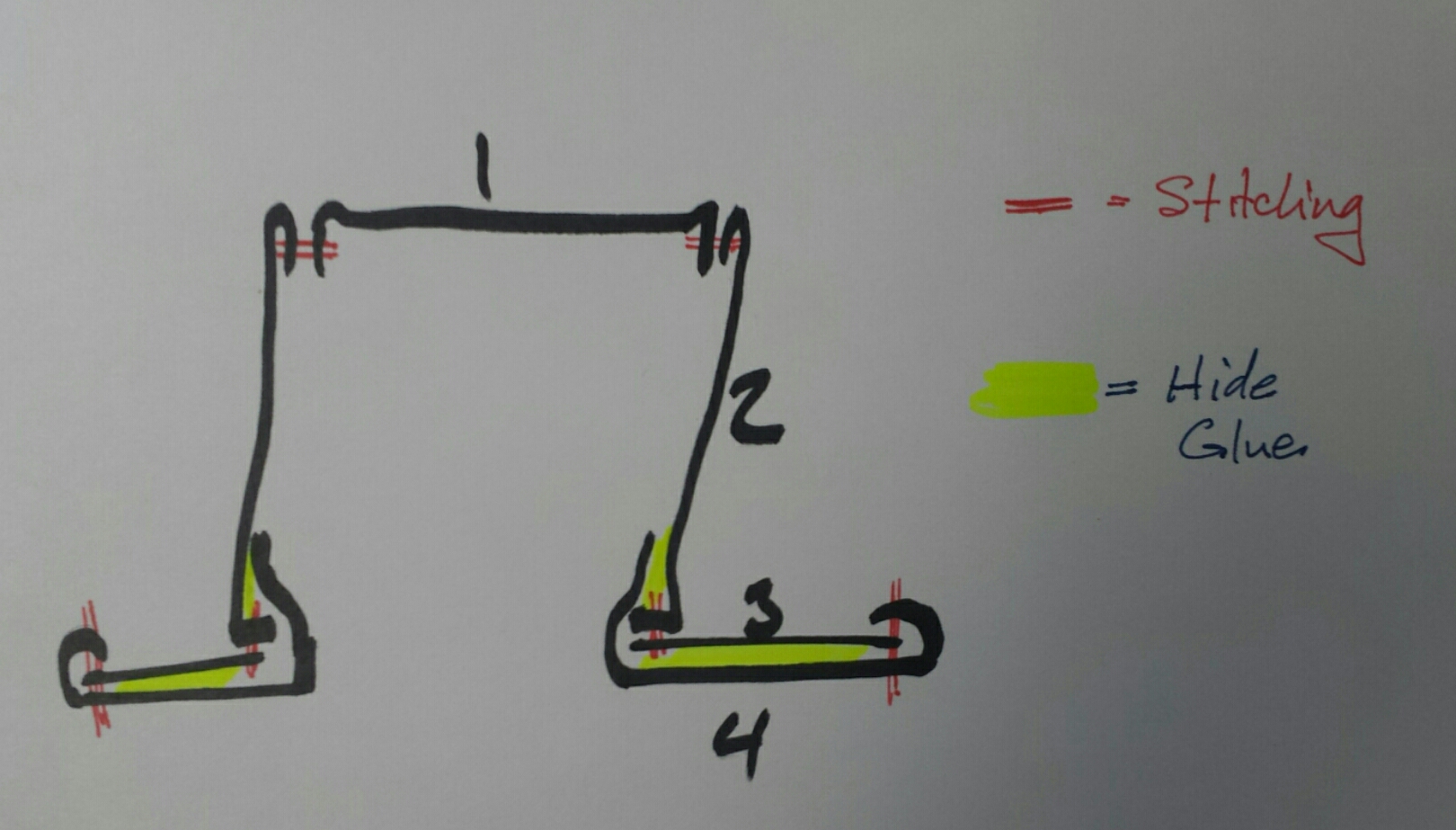The image is a hand-drawn diagram featuring measurements, annotations, and color-coded sections, all depicted on a white piece of paper. The central shape in the diagram is a square missing its bottom side. The remaining two vertical sides of the square are marked by thick black lines. Centered at the top of the square, a black marker indicates the number "1." On the right vertical line of the square, another black marker number "2" is written. 

Just below the missing bottom side of the square, two horizontal lines extend to the right. The upper horizontal line is labeled with the number "3," and the bottom horizontal line is marked with the number "4." Both horizontal lines are shaded in yellow, indicating a specific material used in this section.

The four corners of the square are accentuated by pairs of red marker lines, which are annotated as "stitching" along the sides. Additionally, the areas shaded in yellow are labeled as "hide glue," suggesting that these sections are bonded using this adhesive.

Although the function of this diagram is not explicitly stated within the drawing, it appears to be a detailed representation of various structural elements, utilizing color and numbering for clarity.